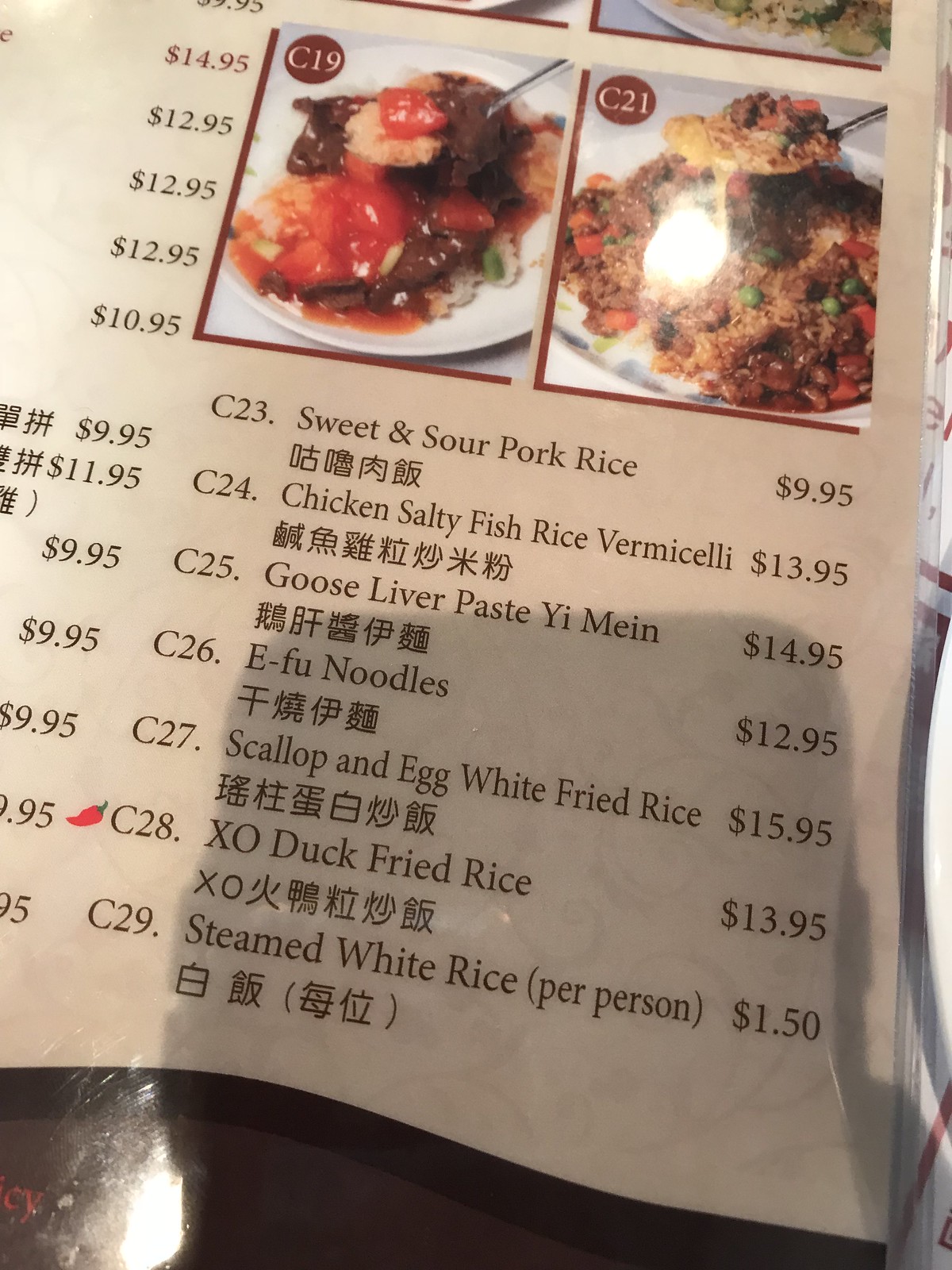The vertically rectangular photograph captures a slightly angled view of the bottom right portion of a restaurant menu on a light tan background. Dominating the upper section of the frame, two square images of different dishes are positioned side by side, providing a visual preview of the offerings. Below these images, a column lists various menu items, each accompanied by a number and price. The dishes and their corresponding prices are as follows: C23 Sweet and Sour Pork Rice at $9.95, C24 Chicken Salty Fish Rice Vermicelli, C25 Goose Liver Paste, C26 Yi Fu Noodles, C27 Scallop and Egg White Fried Rice, C28 Zhou Duck Fried Rice, and C29 Steamed White Rice per person. Beneath the English names of each dish, there are symbols written in either Chinese or Japanese, adding an authentic touch to the menu.